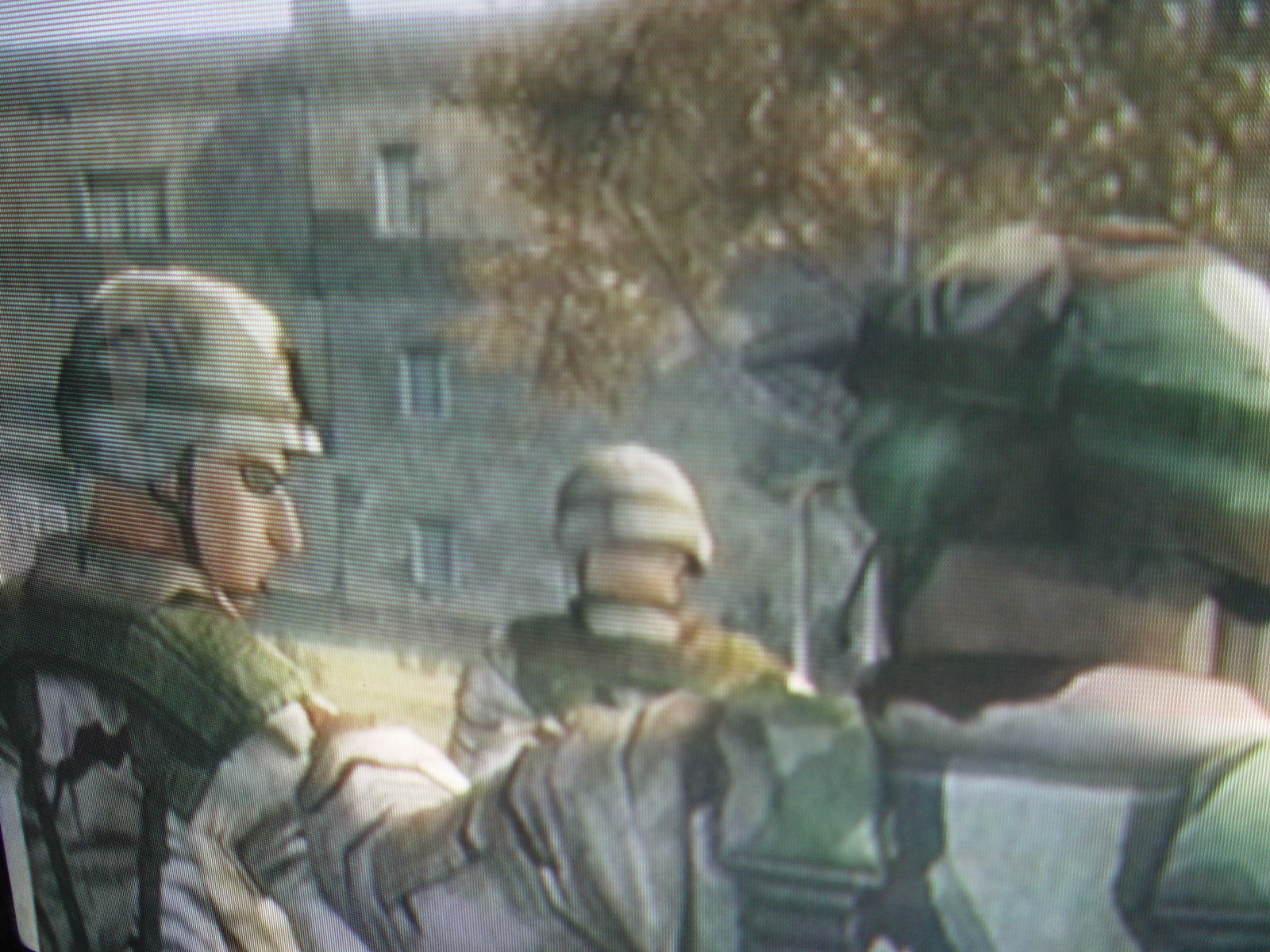The image depicts three soldiers in army fatigues and helmets, viewed from behind. The soldier on the left has small glasses and a camouflage helmet with a strap under his chin, and his distinct down-pointing nose is visible. His left hand is placed on the shoulder of the soldier on the right, who has a very short haircut and seems to be looking to the left with a serious expression. Both soldiers have white skin, emphasizing their camaraderie. In front of them by a few feet, there is a third soldier with a backpack, also in camouflage with a green helmet. They appear to be walking together towards a three-story brick apartment building, characterized by its windows and pillars, with a large tree in front. The scene has a matte, computerized texture giving it a simulated appearance.